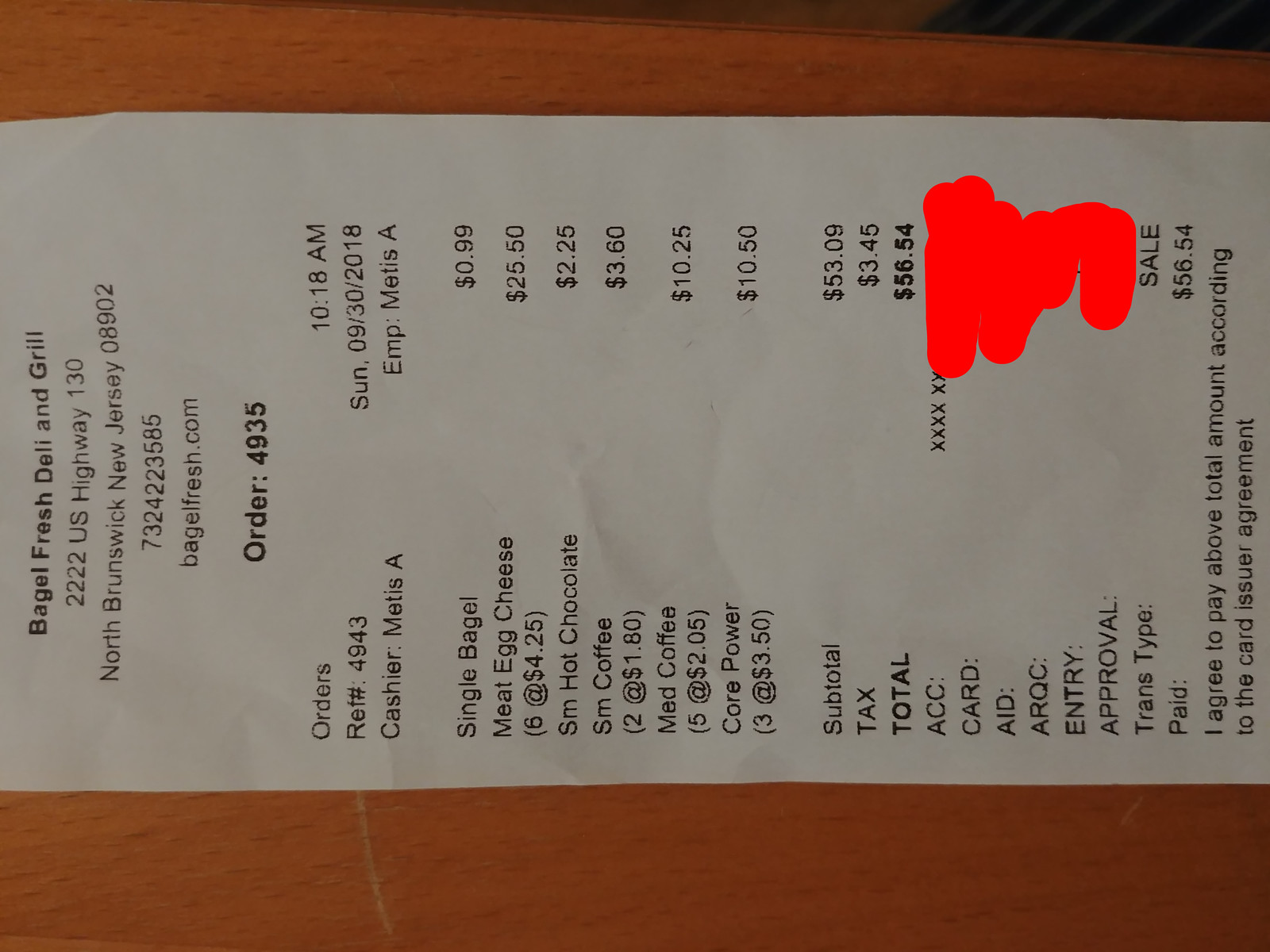The image displays a rectangular-shaped receipt placed horizontally from left to right on a light brown wooden surface. The receipt, made of white paper, is printed with black text consisting of various letters and numbers. At the very top, the heading reads "Bagel Fresh Deli and Grill," followed by the establishment's address, phone number, and website. Below this heading, bold text highlights "Order Number 4935." Further down, the receipt lists the cashier's name, the date, and the time of the purchase.

The purchased items are enumerated clearly: single bagel, meat, egg, and cheese, small hot chocolate, small coffee, medium coffee, and "Cora Power." The total amount spent is $56.54, which is attributed to the purchase of five medium coffees, two small coffees, and six meat, egg, and cheese sandwiches. A notable feature is a red scribble located on the right side of the receipt, seemingly over the cashier's or patron's name. The entire setup rests on a light brown wooden table or desk, giving the scene a casual ambiance.